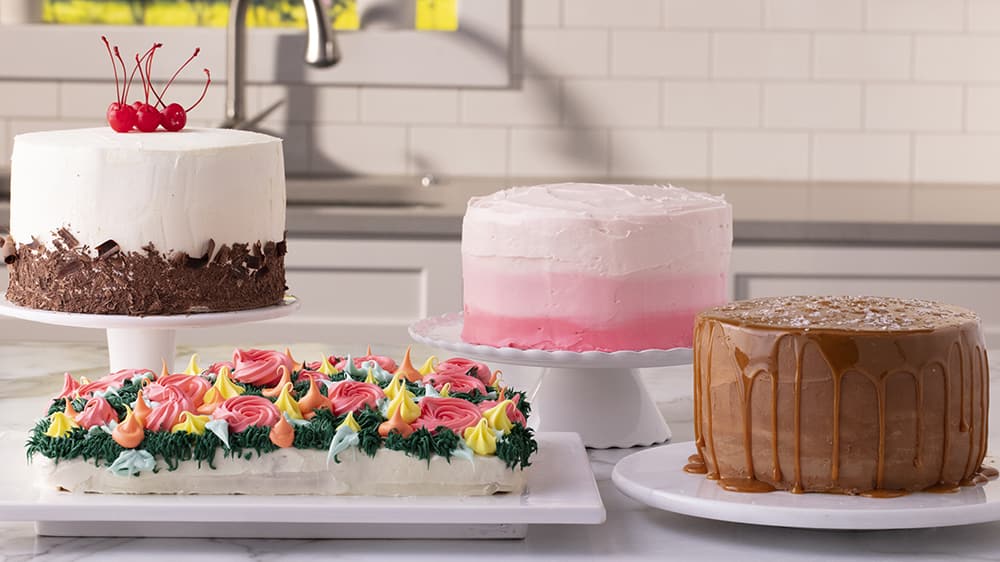This photograph depicts a kitchen scene showcasing an array of four beautifully decorated cakes on a white marble countertop. Against a backdrop of a pale pink backsplash and a kitchen counter with a sink and a window above, the vibrant cakes take center stage. 

From left to right, the first cake is a round creation perched on a tall white cake stand. It features pristine white frosting adorned with chocolate sprinkles along the bottom rim and crowned with approximately three to six cherries on top. The second cake, a rectangular sheet cake, rests on a low platform. Its surface is intricately decorated with swirls of pink, green, and white frosting designed to resemble roses and grass-like elements. 

Next, a striking gradient cake sits on a medium-height white cake stand. This round cake transitions from white frosting at the top to a hot pink base, creating an eye-catching ombré effect. Finally, the fourth cake is a decadent round chocolate cake drizzled with caramel or chocolate ganache, causing mouthwatering drips down its sides. Each cake is displayed on a white plate or stand, emphasizing their detailed decoration and adding to the overall elegance of the setting.